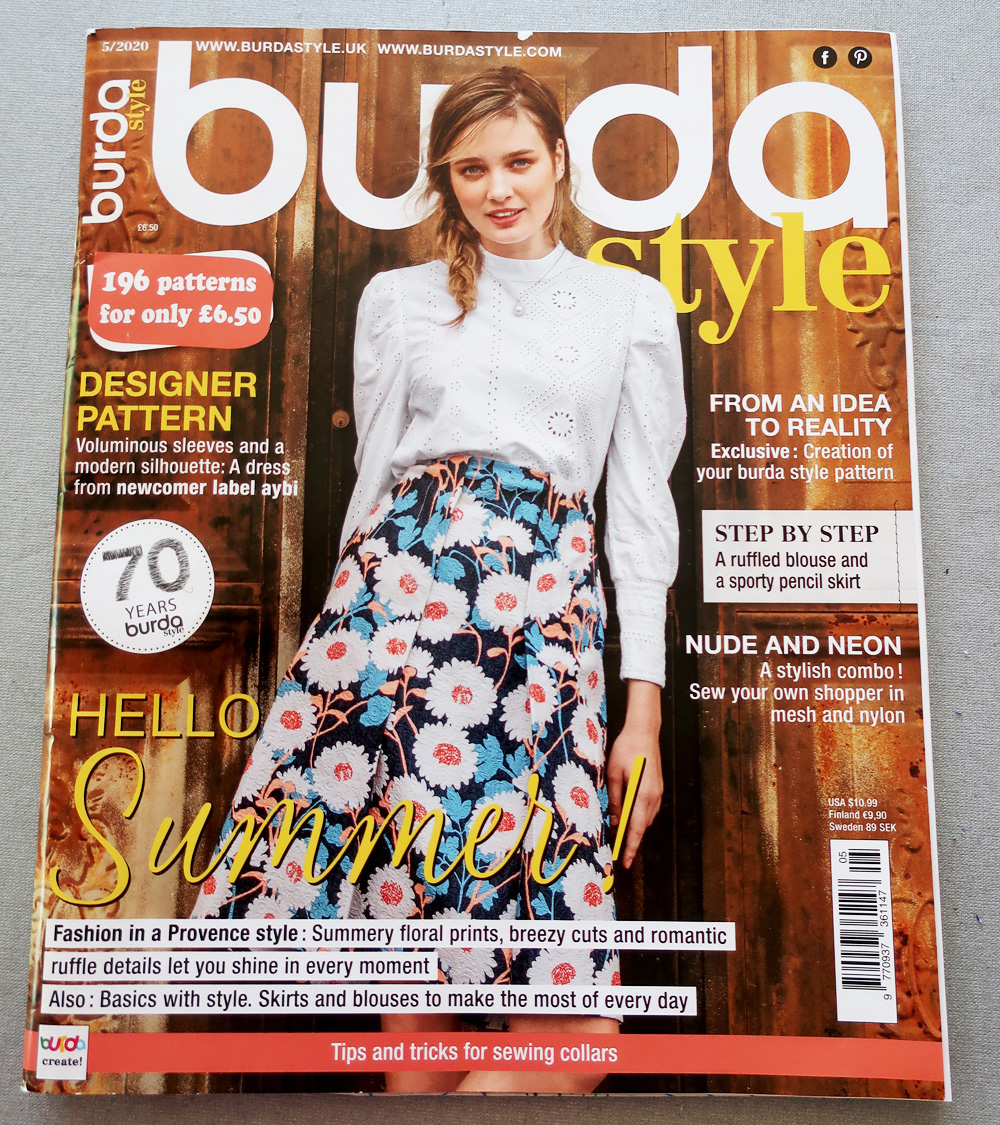The cover of Burda Style magazine features a fashion-forward young model posed against a backdrop of intricate woodwork paneling. The model, whose blondish brown hair is styled in a braid gracefully draped over her right shoulder, is dressed in a chic ensemble comprising a white, long-sleeved blouse with lace sections and a striking floral-printed skirt. The skirt is adorned with an eye-catching pattern of light blue leaves and white flowers, each boasting a distinct peachish-reddish center, all set against a dark blue background. Her pose is relaxed, with her left leg slightly crossed over the other, adding to her casual yet elegant demeanor.

The magazine title "Burda Style" is prominently displayed, with "Burda" in large white lowercase letters and "Style" offset to the right in a classic yellow font. The cover is adorned with vibrant text, the most prominent of which declares "HELLO SUMMER!" with 'Hello' in bold yellow and 'Summer!' in a playful cursive script, exuding a warm seasonal greeting. 

Across the cover, various blurbs and articles catch the reader's eye: "From an Idea to Reality: Exclusive Creation of Your Burda Style Pattern," "Step by Step: A Ruffled Blouse and a Sporty Pencil Skirt," "Nude and Neon: A Stylish Combo," and "Sew Your Own Shopper in Mesh and Nylon." A special feature denoting "70 Years of Burda" is also highlighted in a prominent circle, reflecting the magazine’s rich history. At the top, two website links, www.burdastyle.uk and www.burdastyle.com, provide additional resources for readers. Finally, a noteworthy mention cites a "Designer Pattern: Voluminous Sleeves and a Modern Silhouette, a Dress from Newcomer Label AYBI," offering fashion enthusiasts fresh inspiration.